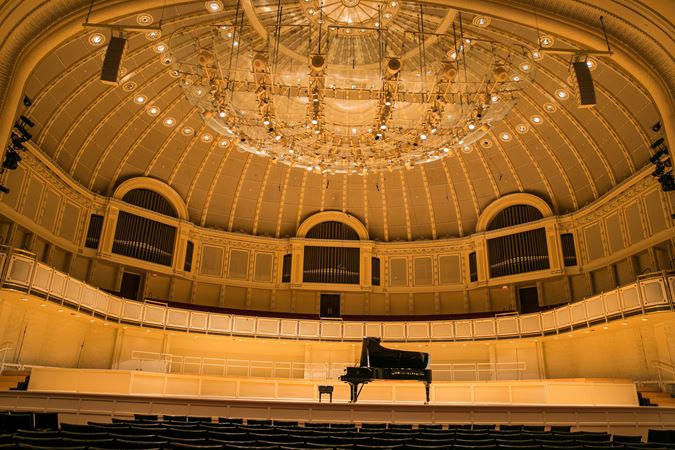The image depicts the interior of an elegant performance center, reminiscent of an amphitheater designed for opera or theatrical plays. The ceiling boasts an oval-shaped dome, adorned with circular lights arranged in a pattern that mimics an elaborate chandelier, lending a luxurious ambiance to the space. At the center of the stage stands a grand black piano, accompanied by a matching stool for the pianist. The first few rows of seating are visible, with the backs of the seats also in black, creating a cohesive color scheme. Additionally, staircases on both the lower right and left sides lead up to the stage, completing the sophisticated and inviting atmosphere of this refined venue.